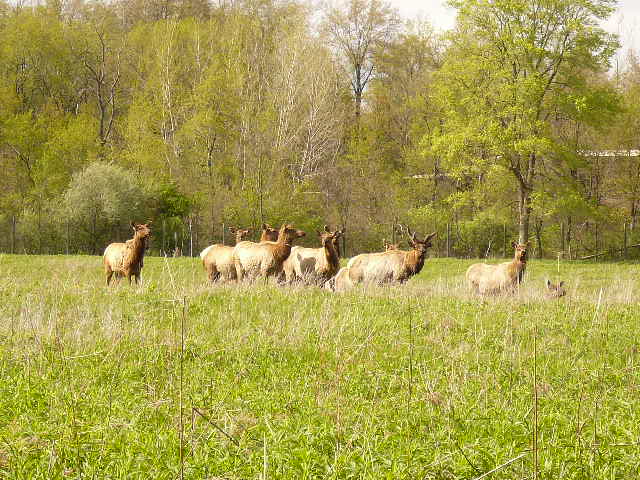The photograph captures a serene outdoor scene taken during the daytime in bright light, displaying a picturesque wilderness setting. In the center of the image, nestled in a broad, unkempt field of tall grass, a herd of approximately ten elk is moving gracefully from left center to right center. The elk are predominantly light brown with darker brown fur around their heads and necks, resembling the coloration typically seen in fawn. 

The animals are depicted in profile, with their erect ears and camel-like necks, though notably, the necks are shorter than that of camels. Most of the elk do not have antlers, suggesting they are females or juveniles; however, on the right side of the image, a larger elk with a full rack of antlers stands prominently. In front of this antlered elk, a smaller antler-less deer and a juvenile are partially nestled in the tall grass, only their heads visible above the foliage. 

The background of the image is dominated by a dense forest of tall, green-leaved trees, under a canopy of light white sky peeking through. The photograph captures the elk group slightly out of focus due to the distance at which it was taken, adding a dreamy quality to the natural scene. Together, the elks and the verdant forest create a tranquil and majestic portrayal of wilderness life.